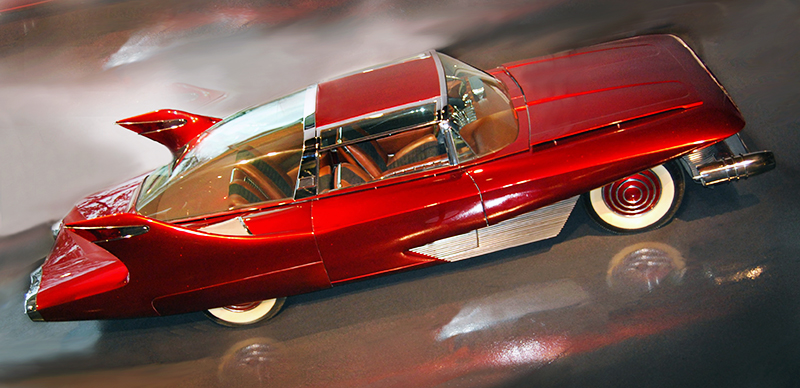The image showcases a highly detailed toy sports car with a candy apple red body and an old-school design. Prominent red fins extend from the back, adding to its classic aesthetic. The car features two doors but includes rear seats, which are visible through the windows and are upholstered in red and black. Its distinctive white-walled wheels have swirly red centers accented with silver parts, and there are dual exhaust pipes on both the left and right sides, also silver in color. The top of the car includes a section that is silver with a red part in the middle that appears to open up. The toy car is resting on a shiny gray surface, which reflects its image, contributing to the overall stylish and captivating appearance.